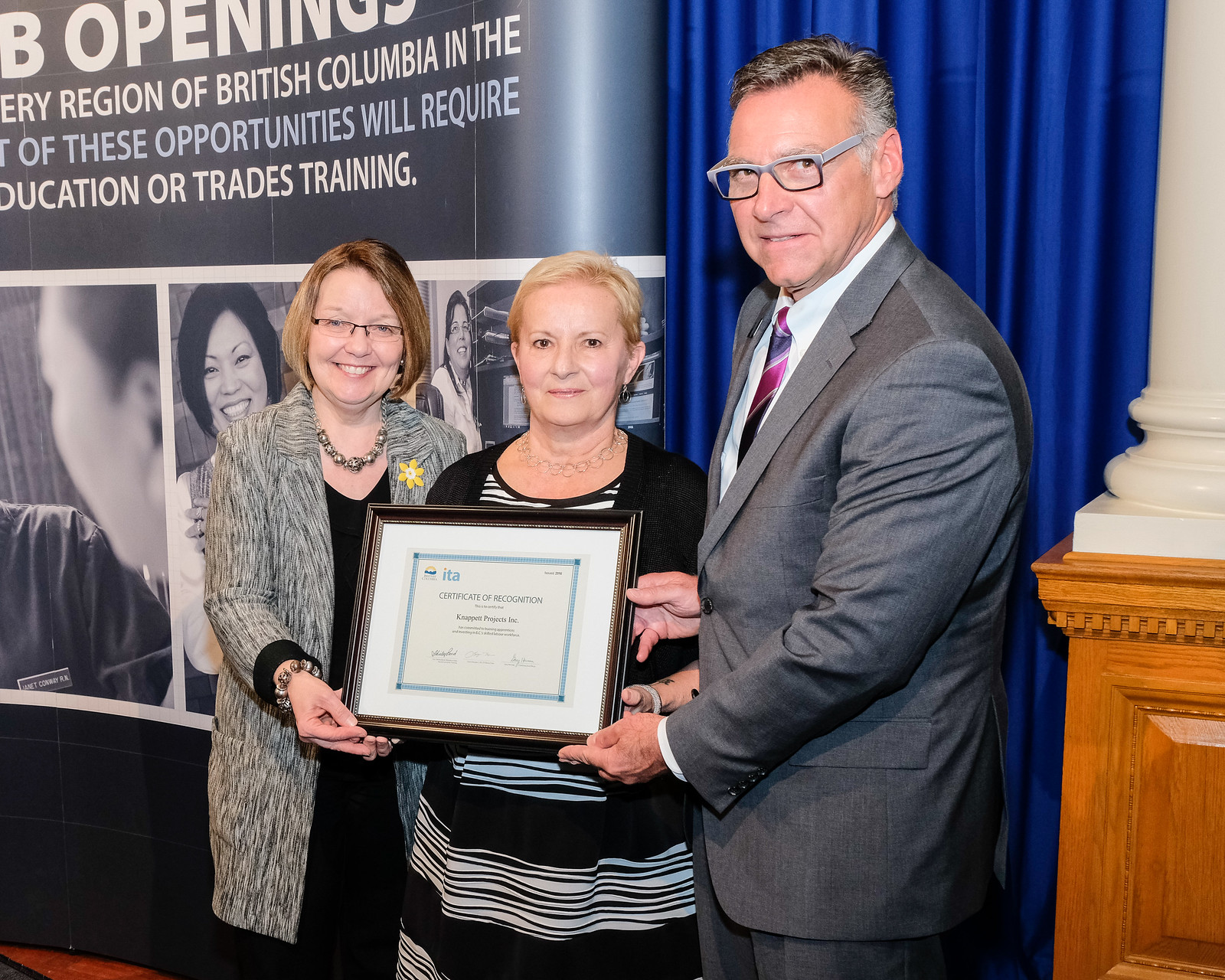The image depicts three elderly Caucasian adults standing in a conference-like setting, proudly holding a framed Certificate of Recognition. In the center stands a blonde-haired woman with a pixie cut, dressed in a black and white striped dress paired with a black cardigan. To her right is a gray-haired man wearing a gray suit with a striped tie and gray glasses, noticeably taller than the women. On her left is a brunette woman with a light-colored bob haircut, clad in a white, black, and gray blazer with glasses. All three individuals are well-dressed and smiling, exuding a sense of accomplishment. Behind them, the backdrop features a blue and dark gray banner with text that partially reads, "Openings, Region of British Columbia," and mentions opportunities requiring education or trades training, suggesting a seminar or professional event. The certificate they hold has a black frame, white matting, and a light-colored background with the text "Certificate of Recognition, Something Projects Inc." and an ITA logo in the upper corner. The overall setting and attire of the individuals suggest a formal recognition at a trades or educational event.